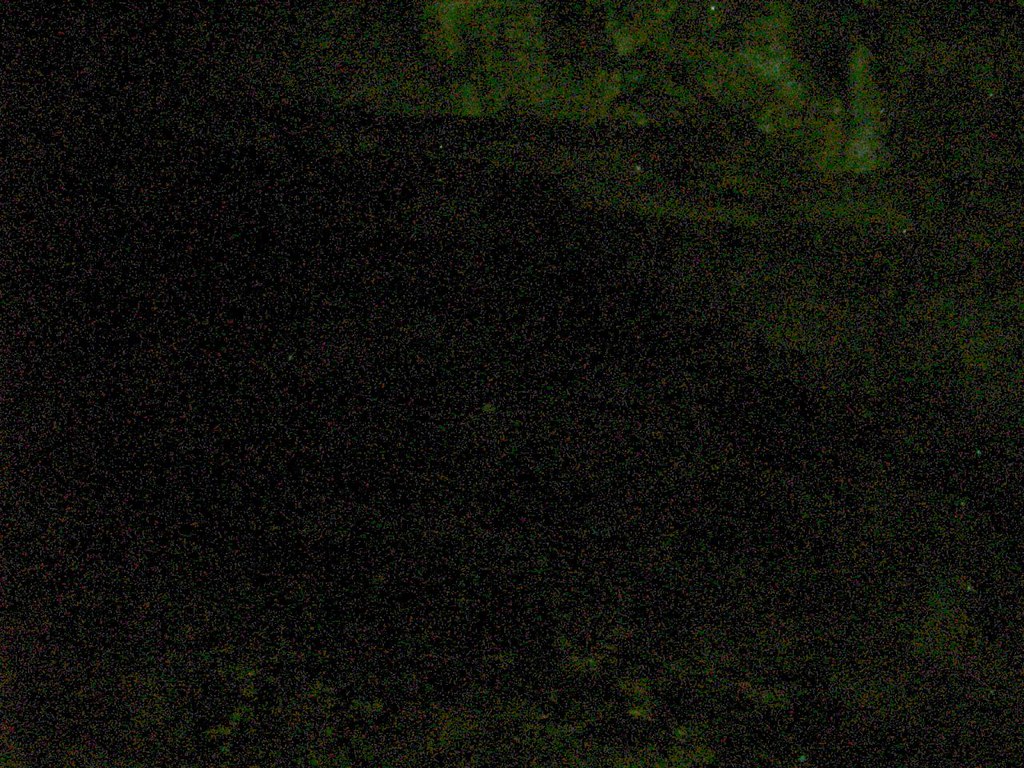The image showcases a heavily textured and grainy scene that is challenging to decipher. The predominant color palette is overwhelmingly dark, with deep, shadowy hues enveloping most of the image. Towards the top, there's a noticeable shift to a lighter green shade, although the details remain indistinct. The bottom of the image continues with the dark theme, contributing to the overall obscurity. The visual noise and extreme graininess make it difficult to determine the exact subject matter, lending an enigmatic quality to the image.